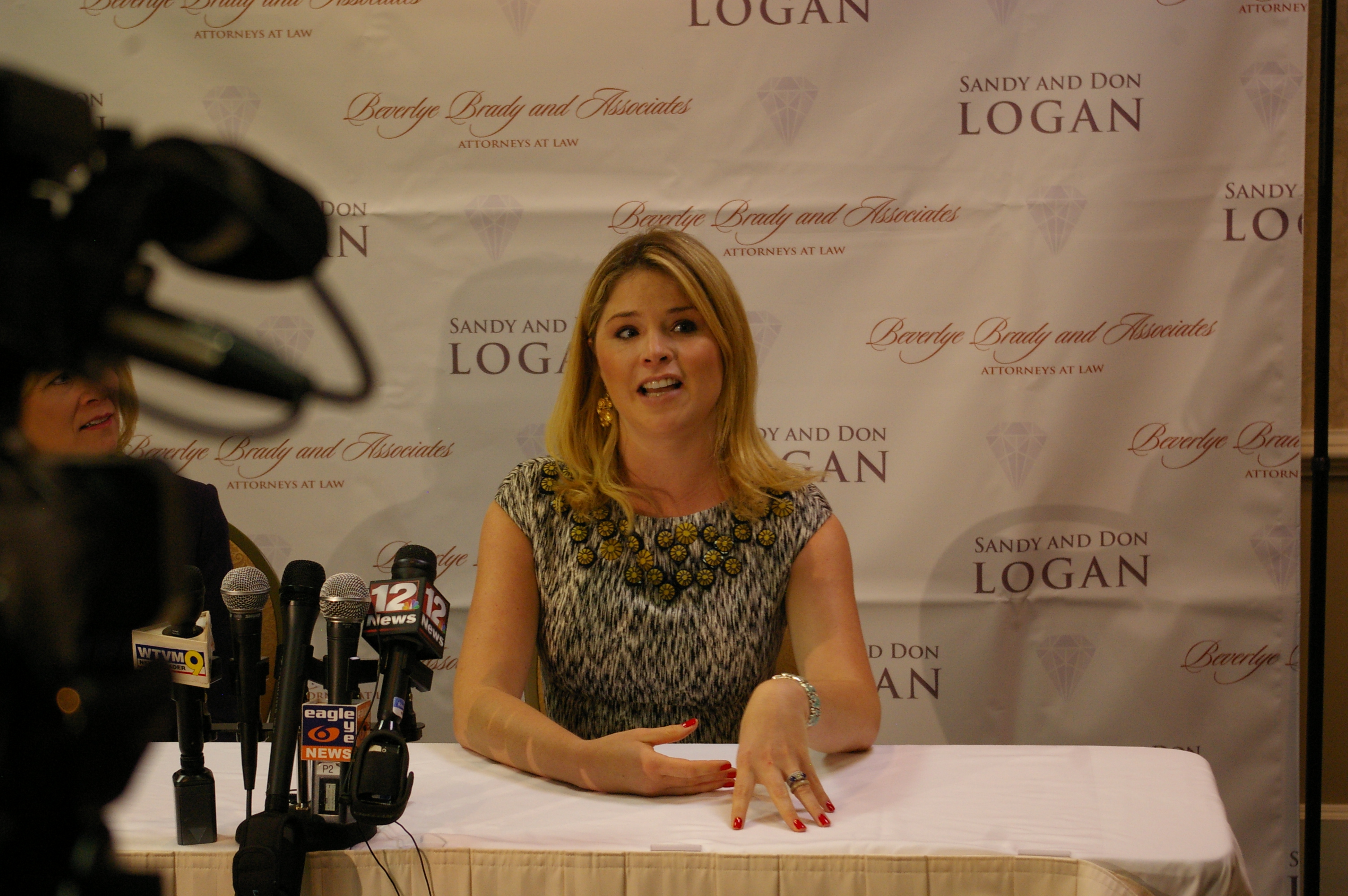In this photo, Jenna Bush, one of the daughters of George W. Bush and Laura Bush, is seated at a table, likely participating in a press conference or interview. The table, covered with a white cloth, is adorned with an array of five microphones positioned in front of her. She is situated in a setting that resembles a conference room or ballroom, evident from the indoor backdrop.

Jenna is donned in a spring-like, very short-sleeved dress that appears to be blue and white with a pattern that could be described as tie-dye with circles. These circles, which mimic flowers, are arranged in a way that resembles a cross-body sash, evoking the look of a Girl Scout sash. She is accessorized with a golden earring visible on her right ear, a shiny metallic bracelet, red fingernails, and a ring on her left ring finger. Her blonde hair frames her face as she speaks with her mouth open, likely mid-conversation.

On her left, another woman is visible, possibly engaged in the dialogue. The background features a sign with two logos, reading "Beverly Brady and Associates Attorneys at Law" and "Sandy and Don Logan," set against a white backdrop. The setting is further accented by a camera on the far left, aimed at Jenna, capturing the moment.